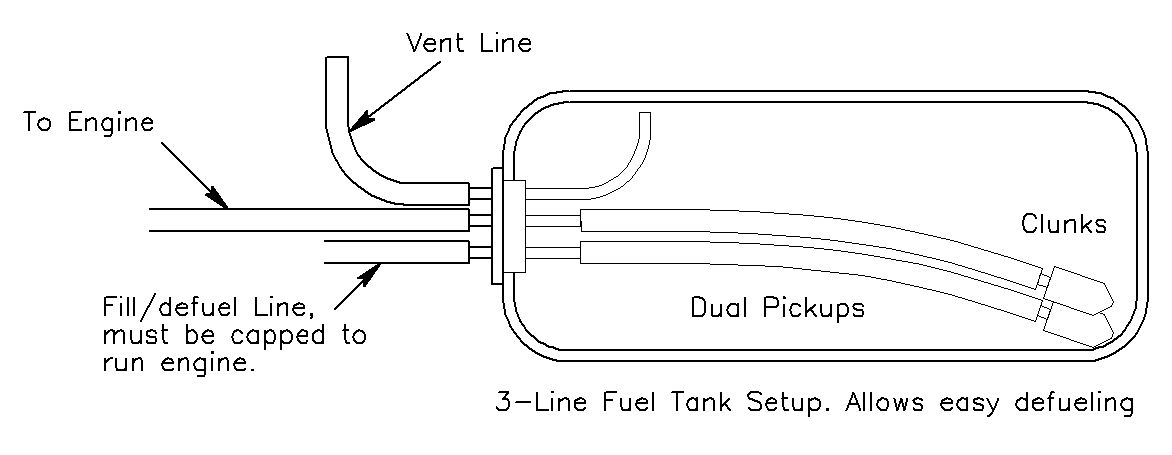The image is a black and white technical line drawing that illustrates a fuel tank system setup. The central focus is a horizontally elongated, rounded-edge rectangular chamber intricately detailed with various tubes. 

On the top left, a tube labeled "vent line" bends upward at a 90-degree angle, indicating its function in venting. Below this, a long straight tube labeled "to engine" indicates the fuel's path to the engine. The lowest tube on the left is labeled "fill/defuel line must be capped to run engine," highlighting its role in both filling and defueling the tank, with an important note about operation.

Inside the chamber, two smaller tubes are labeled "dual pickups," and their ends, equipped with weighted elements known as "clunks," ensure that the fuel lines remain submerged in fuel at all times. The diagram is adorned with thin black lines and arrows pointing to significant components. The layout features clean, sans-serif font labels, ensuring clarity and precision. At the bottom of the image, a caption reads, "three-line fuel tank setup allows easy defueling," summarizing the functionality and convenience of the system depicted.